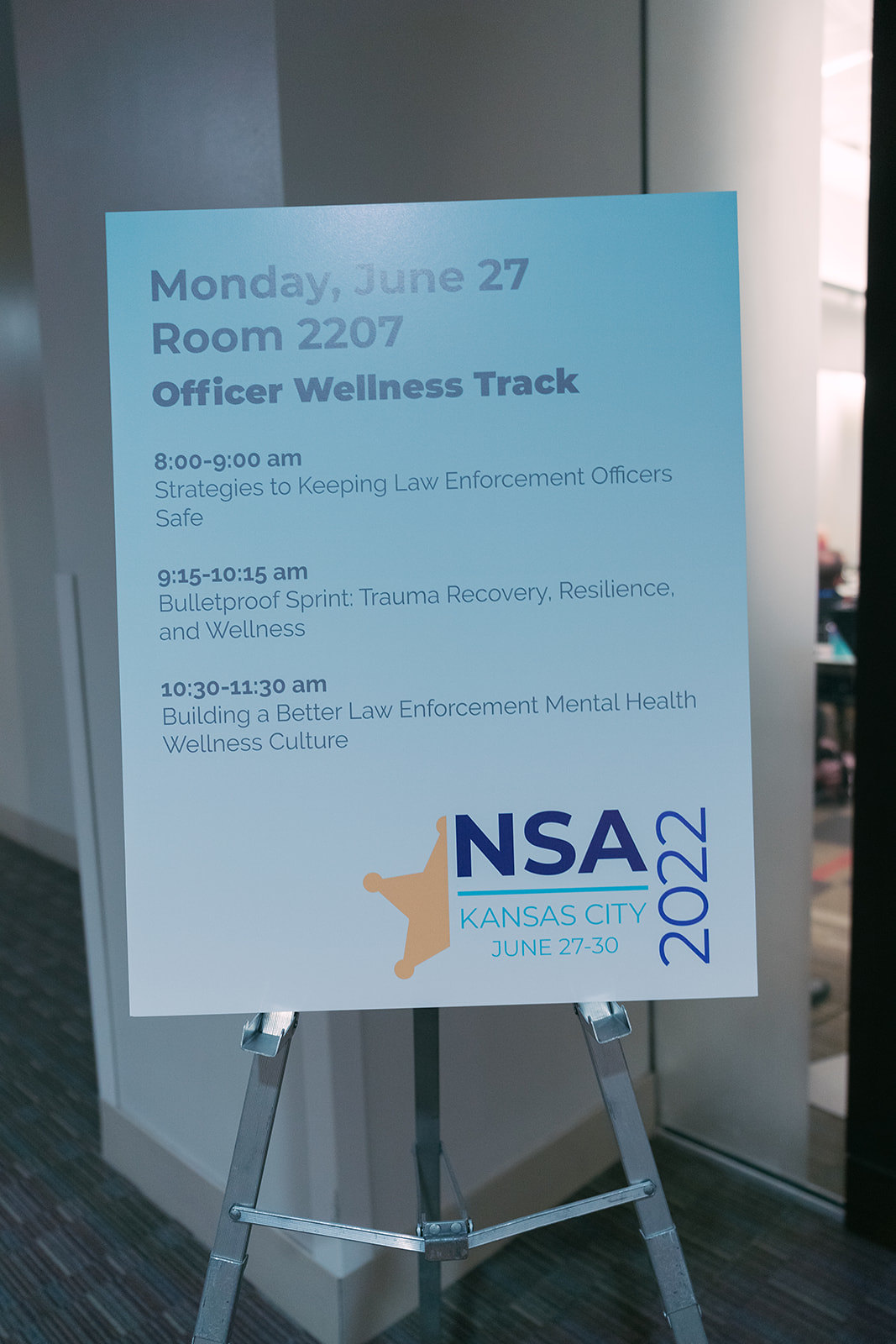This image features a prominently placed sign on a sleek, silver pedestal. The background reveals a conference setting with grayish-green carpet and white walls, along with visible columns and a partial view of a room to the right. The sign, centered in the image, details the "Officer Wellness Track" scheduled for Monday, June 27th in room 2207. It outlines three sessions: "Strategies to Keeping Law Enforcement Officers Safe" from 8 to 9 a.m., "Bulletproof Sprint: Trauma Recovery, Resilience, and Wellness" from 9:15 to 10:15 a.m., and "Building a Better Law Enforcement Mental Health Wellness Culture" from 10:30 to 11:30 a.m. The bottom right corner of the sign features a blue section with the text "NSA 2022 Kansas City" and "June 27th to 30th," along with half of a yellow star. The diverse colors in the image—gray, silver, white, blue, orange, light blue, pink, and red—enhance the indoor conference ambiance.